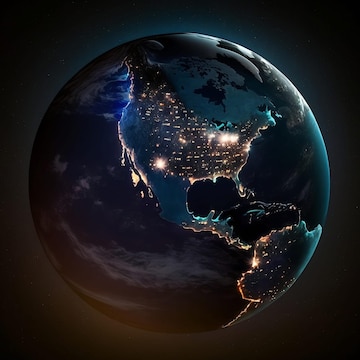This image showcases a detailed, artistic rendering of the Earth primarily focused on North and Central America, with parts of South America visible towards the bottom right. The globe, a shiny orb, features a dark palette with deep blues and blacks representing the oceans and landmasses. The United States is illuminated with numerous white lights, highlighting major areas like Southern California and New York City, while the rest of North America and South America display a mix of darker blue shades and scattered lights. Notably, Canada and Mexico have fewer illuminated areas. Surrounding the Earth is a blue aura, blending into a space background dotted with tiny white stars. A distinct reflection, likely from the moon, appears in the upper right corner, adding to the ethereal quality of the image. The juxtaposition of illuminated lands against the dark oceans and space creates a striking visual contrast, emphasizing the inhabited areas of the globe.